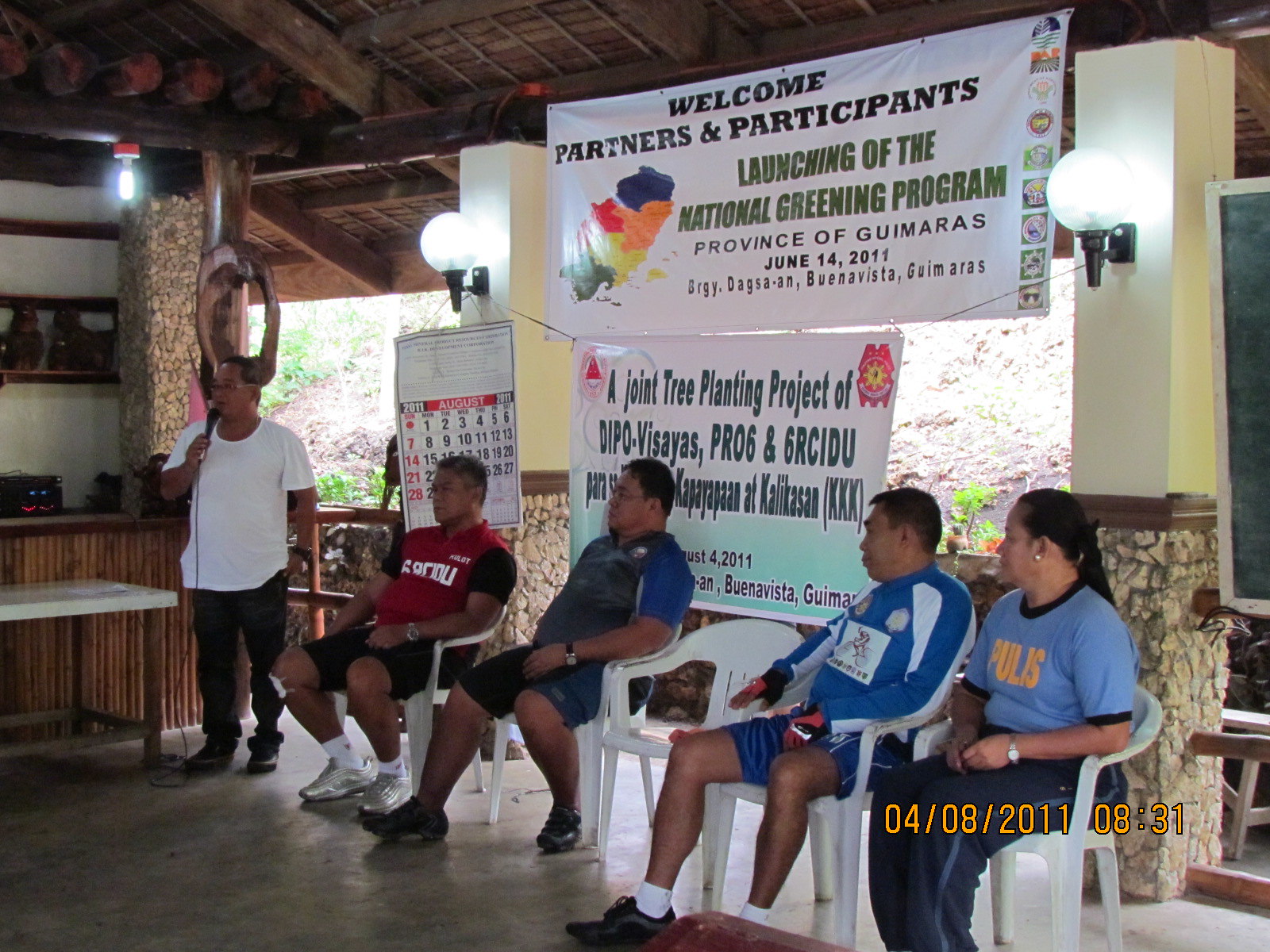In this open-air pavilion characterized by its thatched brown roofing, fluorescent lights, and surrounding greenery, a gathering is underway. The focal point is a man standing at the left edge of the assembly, speaking into a microphone. He has dark hair, glasses, and wears a white t-shirt and dark pants. Seated in a row of white plastic lawn chairs in front of him are four individuals: three men and one woman. They all have dark hair and darker skin tones, suggesting Hispanic or Asian descent. Directly in front of the speaker is a table, and behind him is a bar area.

From left to right, the seated individuals include: a man in a red shirt and black shorts; a man in a gray shirt with black shorts; an empty chair; a man in a blue shirt and blue shorts; and a woman with long dark hair, wearing a light blue shirt and dark pants. They appear to be attentive to the man holding the microphone. Behind them, banners hang prominently, reading “Welcome Partners and Participants, Launching of the National Greening Program, Province of Guemars, June 14, 2011” and “A Joint Tree Planting Project of Dippo, Visases, PR-06, and 6R-CIDU.” Off to the side, there is also a large printed calendar. This detailed scene captures a significant environmental event aimed at promoting tree planting initiatives.